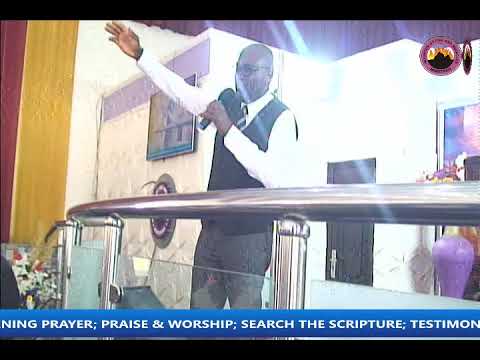The image captures a grainy, overexposed photograph of a TV screen featuring a preacher delivering a sermon. The preacher is a bald black man wearing prescription glasses, a white dress shirt, a striped tie, a black vest, and gray pants. He is holding a microphone in his left hand with his right hand outstretched upward. He stands behind a silver metal railing with glass panels at the bottom. The background reveals white marble walls with glaring lights from above, slightly blurring the screen. To the right, there is a circular logo with a mountain design. On the stage, potted plants and a purple vase are visible. At the bottom of the screen, a blue banner displays the phrases: "Prayer; Praise and Worship; Search the Scripture; Testimony."